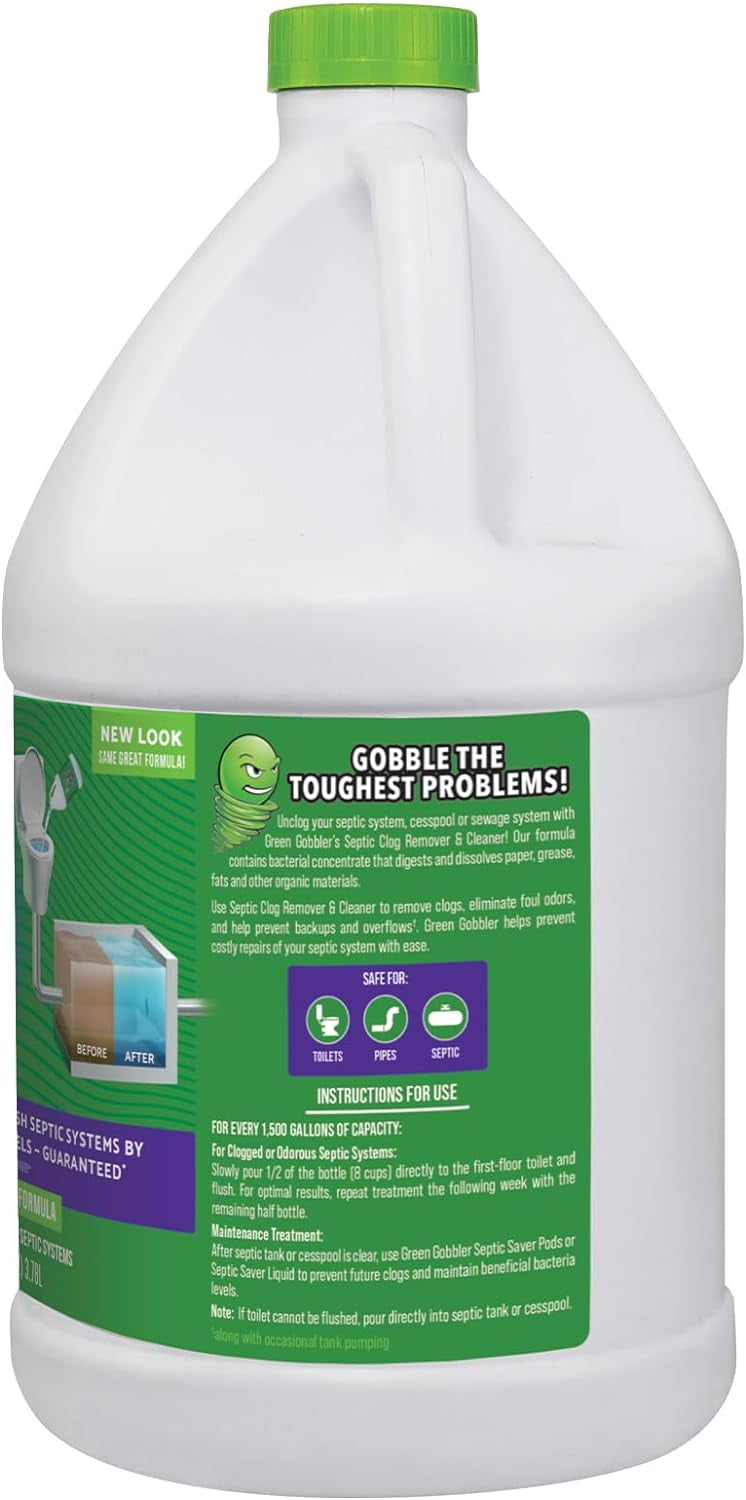The image features a product photo of a gallon-sized white plastic jug designed for the treatment of septic tanks. The jug has an integrated handle at the top and a light lime green screw cap. The label covering the middle section of the jug is green, prominently displaying a bold white text with a black outline that reads, “Gobble the toughest problems!” Below this tagline, smaller white text details the product's use as “Green Gobbler's Septic Clog Remover and Cleaner.”

On the left side of the label, there's a detailed diagram illustrating the efficacy of the product: a drawing shows the jug being poured into a toilet, followed by a depiction of a septic tank with a "before" image of brown water transitioning to an "after" image of crystal blue water, highlighting its cleaning effectiveness.

At the top of the label, it says, “New look, same great formula.” Additionally, a green character with large, spooky eyes and a wide, toothy mouth appears, engulfed by a tornado effect beneath him. The label also includes a purple rectangle featuring three green circles with icons inside: a toilet, a pipe, and a septic tank, signifying that the product is safe for all three.

The back of the jug includes detailed usage instructions: “For every 15,000 gallons of capacity, for clogging or odor of septic system, slowly pour half of the bottle, eight cups, directly into the first-floor toilet and flush. For optimal results, repeat treatment the following week with the remaining half bottle.” It also suggests using Green Gobbler's Septic Saver Pods or Septic Saver liquid for ongoing maintenance to prevent future clogs and maintain beneficial bacteria levels.